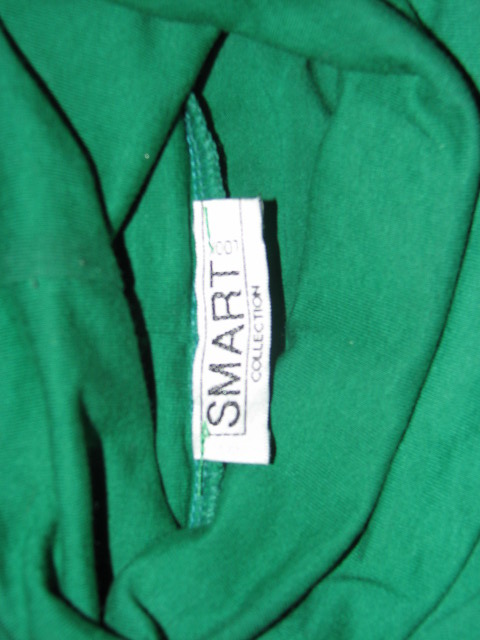The image presents a close-up view of a forest green piece of clothing, showcasing a white tag located centrally on a seam. The tag is meticulously stitched into the green fabric with green thread. The tag prominently features the word "SMART" in large, all-capital black letters, which is enclosed within a black-outline square extending to the top of the tag. Beneath "SMART," in a smaller font and also in black capital letters, the tag reads "COLLECTION." Additionally, there is a lighter inscription reading "001" positioned next to the letter "T" in "SMART." The photograph is zoomed in, making the tag the central focus against the green fabric backdrop, which appears to cover the entire picture. The clothing item seems to be shown inside out, highlighting the seam and stitching details.